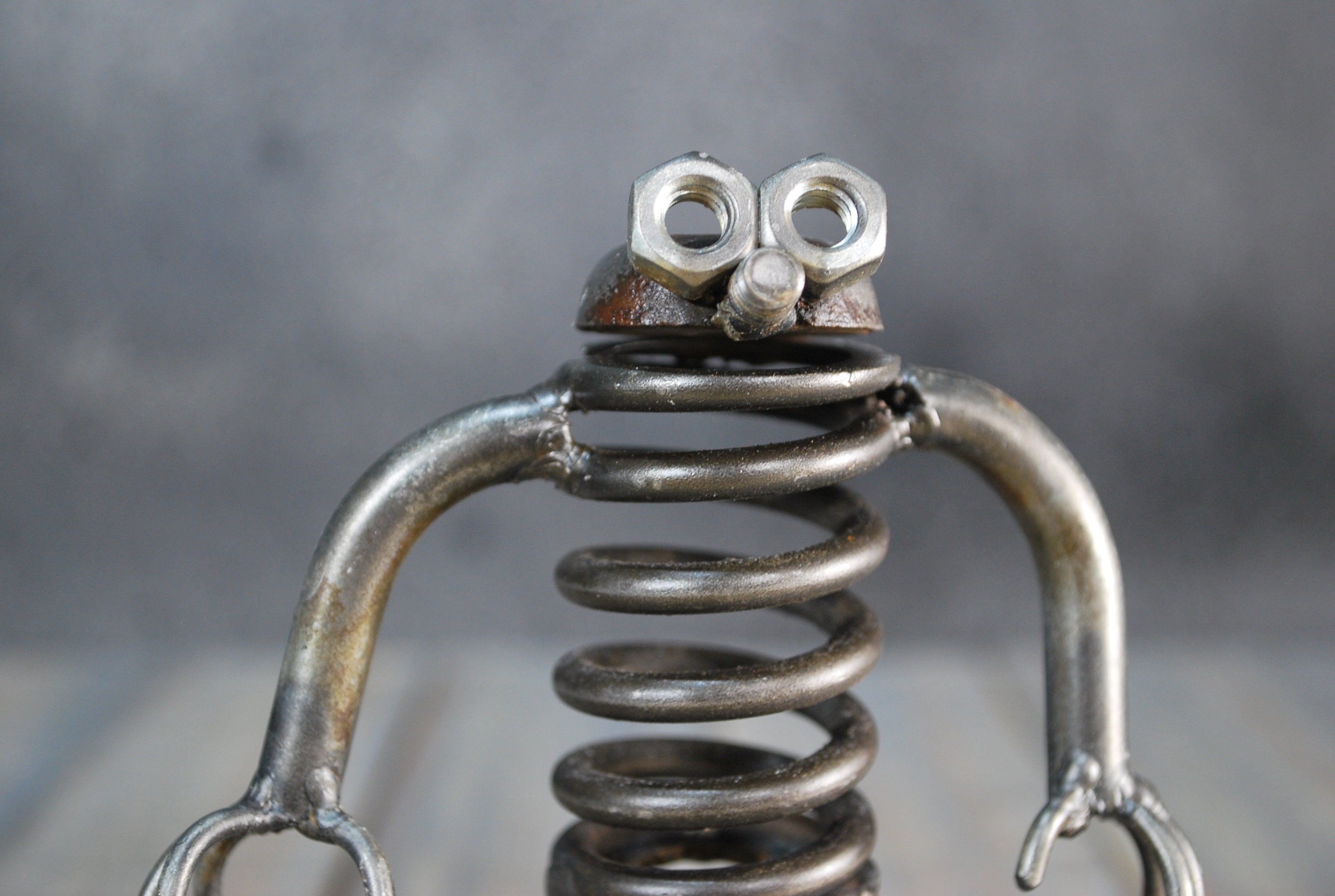This image showcases a charming piece of folk art created by welding various industrial metal parts into a humanoid robot figure. Set against a blurred gray background, this detailed artwork is prominently featured in the foreground, occupying nearly the entire frame. The body of the robot is made from a thick, darkened metal coiled spring, giving it a sturdy and robust appearance. The arms, crafted from thick metal bars, are soldered onto the coil and end in open, slightly bent round links, resembling hands. The head is fashioned from a rusted metal end cap, with two washers serving as eyes and a small tool or screw acting as the nose, projecting a whimsical and creative expression. The design is a testament to the artist's ingenuity in repurposing simple industrial components into an expressive and cohesive figure.